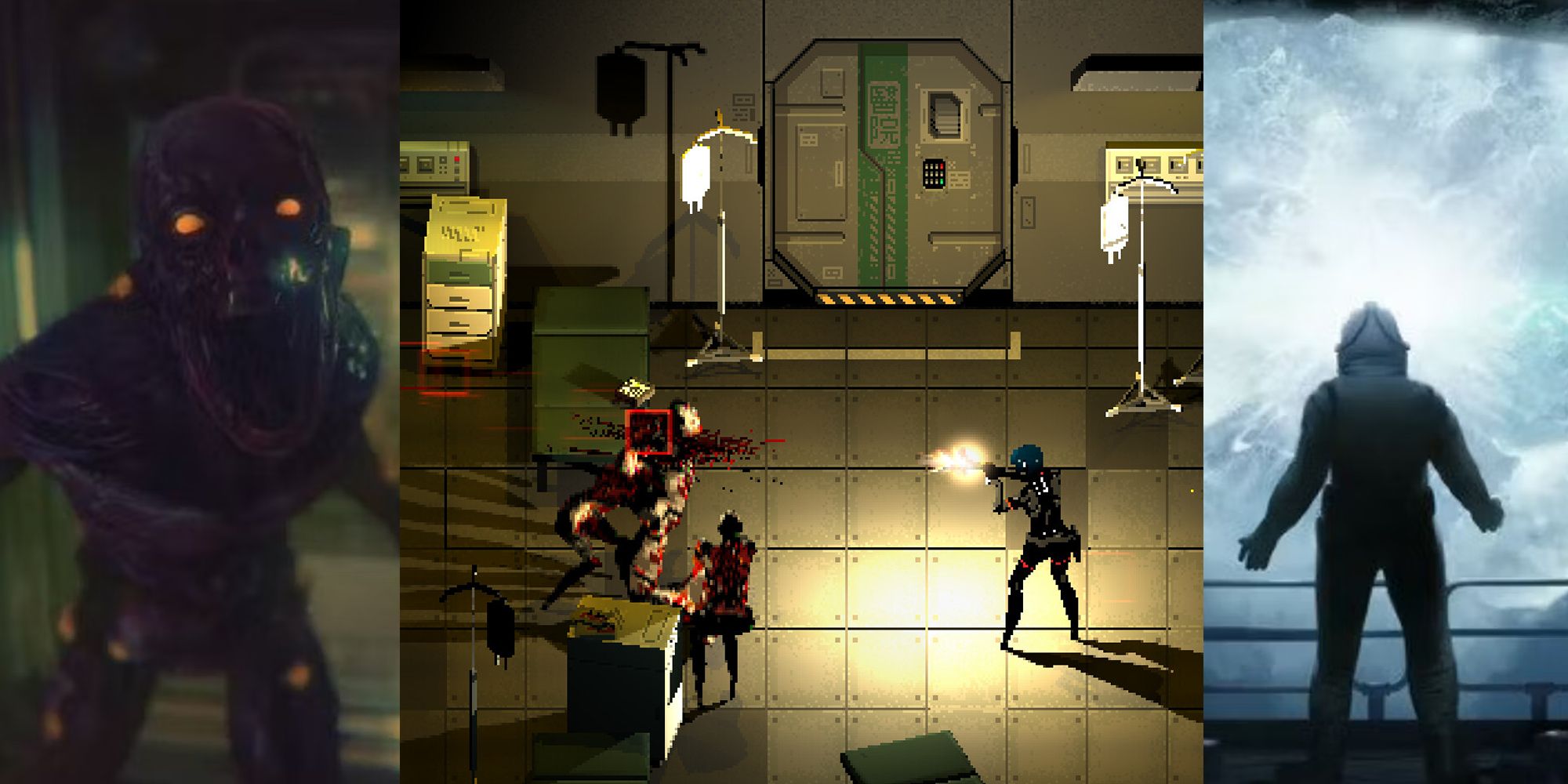The image depicts a collage of three scenes from a video game characterized by its pixel art style and set within a scientific lab or spaceship environment. On the left, a menacing, black metallic skeleton with glowing orange eyes screams directly at the viewer, creating a sense of immediate tension. In the center, a dramatic confrontation unfolds as a character in a dark suit with a blue helmet shoots at a monstrous enemy. Blood can be seen gushing from the creature, suggesting a direct hit, while another figure nearby also seems to be affected. The setting is detailed with tiled metal flooring, an electronic door featuring Japanese or Chinese characters and a keypad, as well as medical equipment like IV poles with glowing saline bags. On the right, a suited figure stands with their back to the camera, observing a radiant burst of light in the sky. This scene is framed by a railing, enhancing the sense of a futuristic or extraterrestrial landscape.